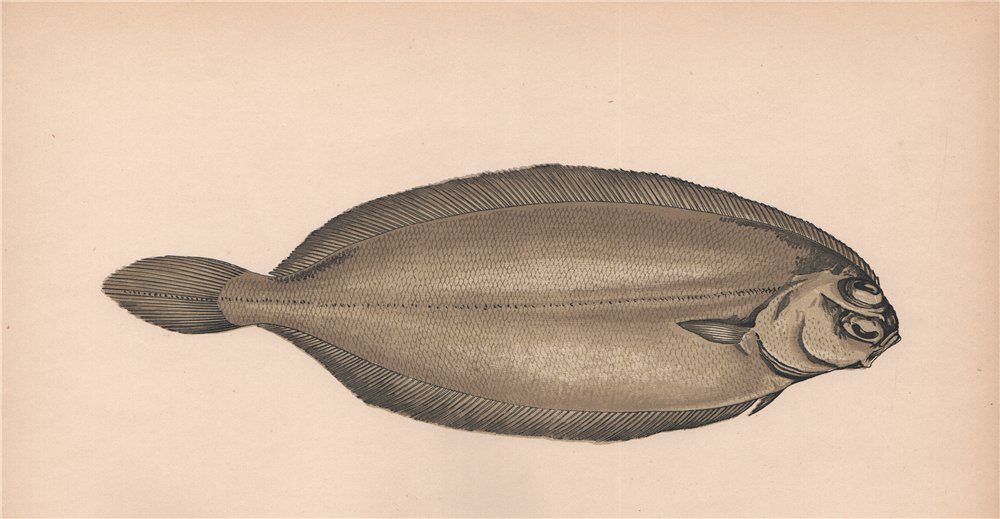The image features a detailed portrayal of an unidentified fish with a bulbous midsection, centered against a solid light tan, almost pinkish background. The fish is primarily brown with blended shades of white and black, exhibiting realistic detailing. Its head has an odd shape with two prominently visible eyes positioned on top, suggesting the image was taken from above. The fish has a round, slightly open mouth directed towards the lower right corner of the frame, and a distinguishing black line stretches from the head to the tail along its back. The upper and lower parts of the fish's body have different textures, and something protrudes from its head. The tail is modest in size, featuring a combination of black, white, and brown stripes. There are no additional elements such as text, numbers, or water in the picture, making the fish the sole focal point of this striking yet peculiar composition.